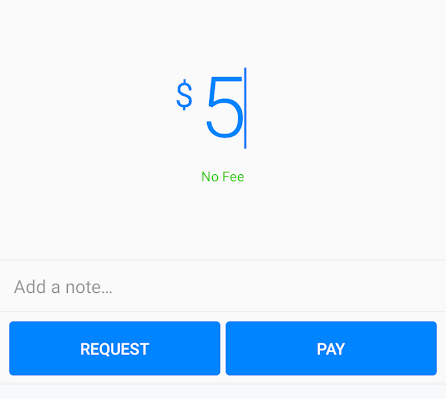This cropped screenshot appears to originate from either a website or an application, specifically designed for monetary transactions. The central focus of the image is a grey square interface. At the top center of this box, there's a blue text indicating a dollar sign followed by a large digit "5", accompanied by a line suggesting an editable field for entering or adjusting the amount. Directly below the amount, green text reads "No Fee". Further down is a section labeled "Add Note," allowing users to include a memo for the recipient of the funds. At the very bottom of the interface, there are two prominent blue buttons; one labeled "Request" and the other "Pay". The overall design closely resembles the interface commonly used on Facebook for sending or requesting money, although no specific branding is visible in this screenshot.